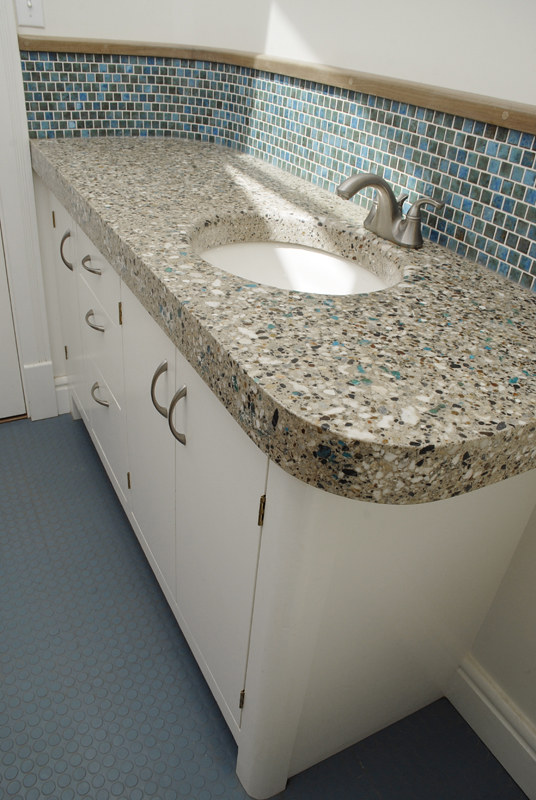A stylish bathroom vanity featuring a diagonal view of a granite countertop showcasing a rich amalgamation of brown, tan, white, and several darker areas, particularly prominent on the front right corner. The perspective runs from bottom right to top left, revealing a white recessed sink set into the countertop. Above the sink is an elegant curved silver faucet. Below the countertop are three cabinet doors and three drawers, each adorned with gold or brown handles, providing ample storage.

The backsplash is adorned with a pattern of small blue and gray tiles, possibly hexagonal or square, adding a splash of color and texture to the space. Topping the tiles is a strip of light brown molding, and above that, a clean white wall extends upward. To the upper left corner of the image, the frame of a door is visible, hinting at the layout of the room. The countertop is pristine and free of any items, suggesting the bathroom is part of a vacant house.